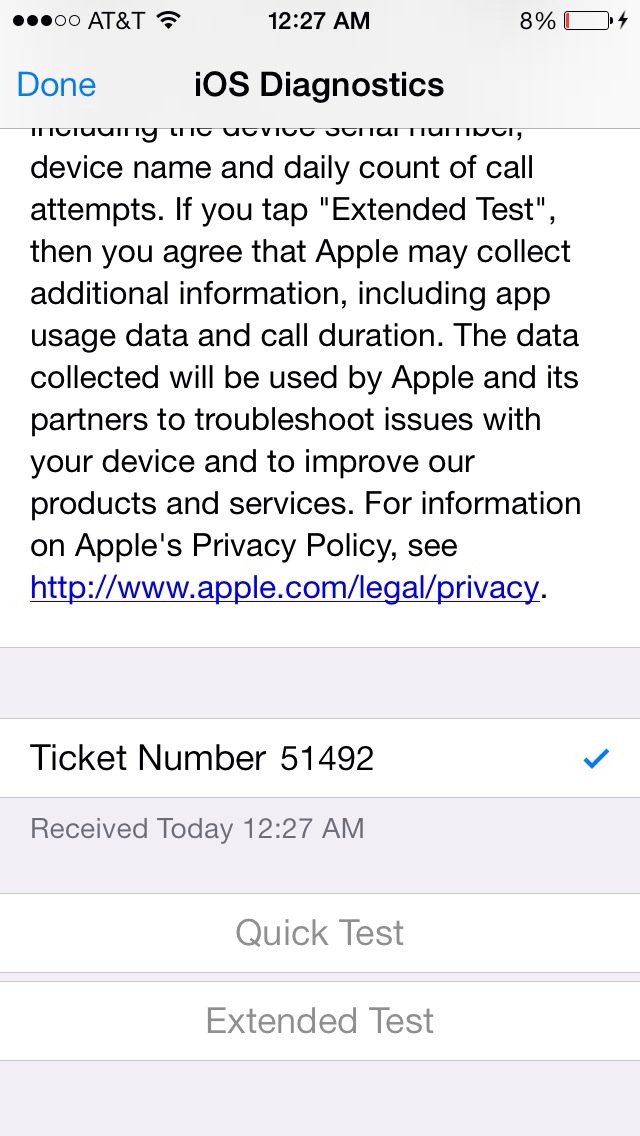This is a detailed screenshot taken on an iPhone, as indicated by the status bar at the top displaying "AT&T," a Wi-Fi signal, "12:27 AM," and "8% battery" being charged. The image captures the iOS Diagnostics screen, identifiable by the title "iOS Diagnostics" at the top and a blue "Done" button, which allows users to exit.

Central to the image is a notification about diagnostic tests. The text explains that tapping "Extended Test" signifies an agreement to let Apple collect additional information, including app usage data and call duration. This data will be utilized by Apple and its partners to troubleshoot device issues and enhance their products and services. A URL to Apple's privacy policy, "apple.com/legal/privacy," is included for more detailed information.

Below this text, there is a section for a support ticket, labeled as "Ticket number 51492" with a blue checkmark next to it, signifying an active or resolved issue. This ticket was received at "12:27 AM." Following this are two buttons: "Quick Test" and "Extended Test," indicating options for further diagnostics. The screenshot’s color scheme and layout align with typical iPhone styling, featuring portrait orientation and a mix of white, gray, and blue elements.